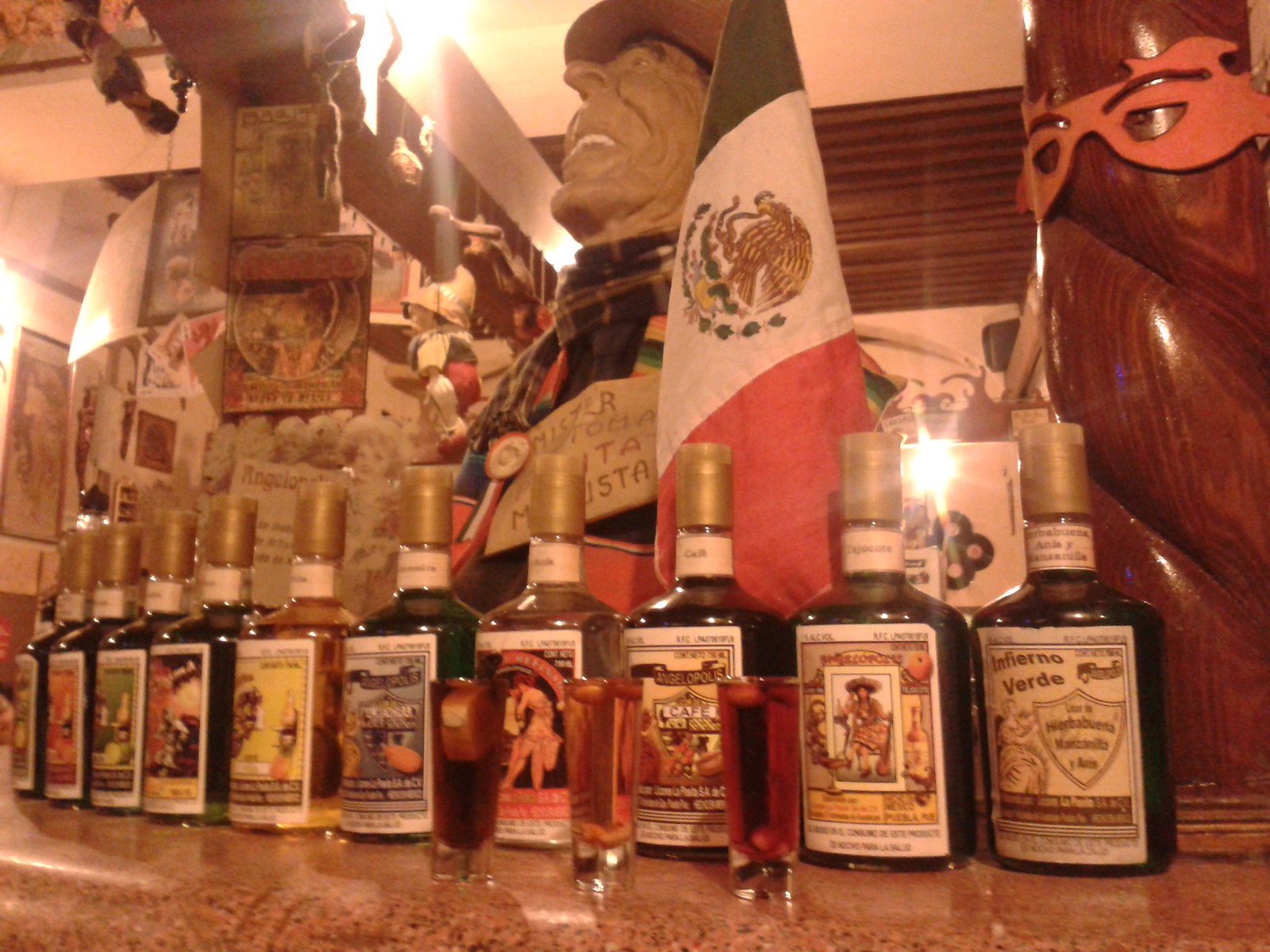This image, taken with artificial lighting that casts an orange-yellowish hue, appears to be inside a bar or tasting room. The setting features a speckled marble countertop, brownish-orange in color, spanning the bottom of the frame. On this counter, a lineup of several identical, large bottles of liquor, each capped with gold and labeled differently, is arranged in a slight semicircle. In the center of this arrangement, three double shot glasses stand side by side, containing reddish, orangish, and very dark brown liquids. Above these bottles, a prominent wooden statue of a cowboy, adorned with a hat and a neck scarf, holds a dark blue, white, and red flag. Additionally, a twisted wooden pillar with a red mask is visible on the right side of the image. The background is decorated with various pictures, postcards, and bar paraphernalia, contributing to the eclectic ambiance.